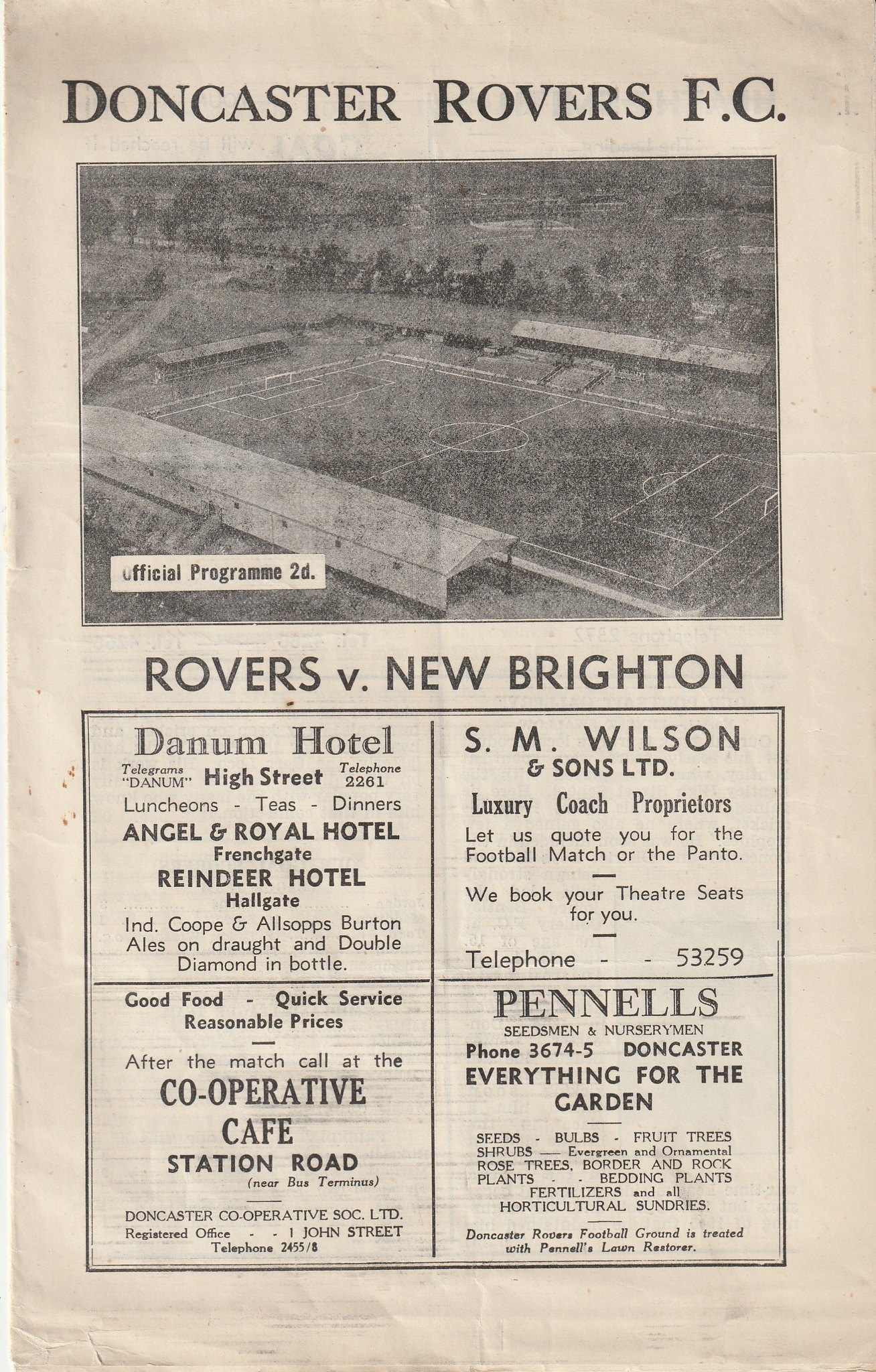This vintage black-and-white image resembles the front cover of an old newspaper or program, dedicated to the Doncaster Rovers Football Club. Across the top in bold, all-caps black text, it proudly states "DONCASTER ROVERS F.C." Directly below is a black and white photograph capturing an empty soccer field with trees and surrounding areas in the background, giving a serene yet nostalgic atmosphere. Positioned on the bottom left of the image, "Official Program 2D" is printed in black text, followed by "Rovers V. New Brighton," indicating an upcoming match. The lower part of the program features a box divided into four smaller advertisements. The top left segment promotes the "Danum Hotel," while the top right highlights "S.M. Wilson and Sons Ltd." The bottom left box advertises "Good Food-Quick Service" with a note on "Reasonable Prices" beneath it, likely referring to a cooperative cafe, and the bottom right square mentions "Pennell's," possibly indicating a garden center or landscape nursery. This image exudes a historical charm and offers a glimpse into past sports culture through its well-preserved advertising and layout.